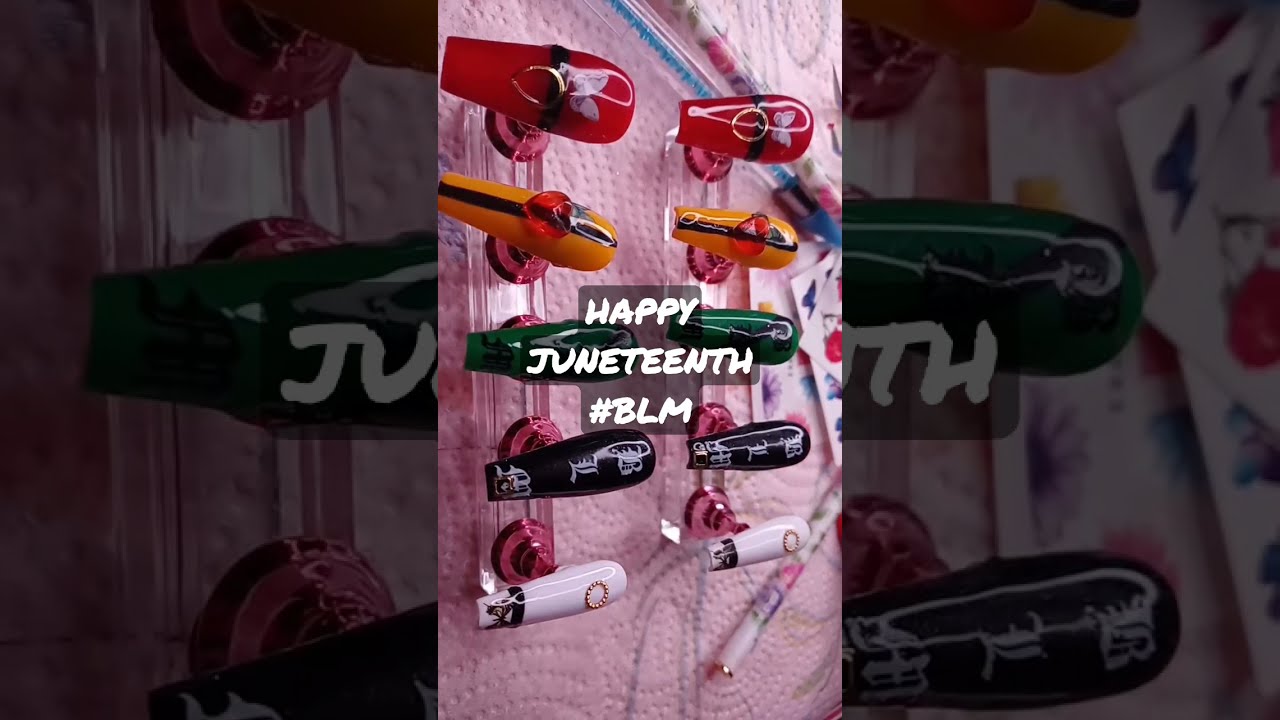The image captures a celebratory ode to Juneteenth, emphasized by vibrant and artistic fingernail designs. At its center, the text "Happy Juneteenth #BLM" in white writing stands prominently. The nails, likely prepared for a social media post on platforms like Facebook or Instagram, exhibit striking diversity and intricate decorations. Arranged in two vertical rows, the nails rest atop a paper towel, typical of those used by nail technicians to catch any drips.

- The top pair of nails are red with a black band and adorned with a single butterfly motif above a gold ring.
- The second pair features yellow nails, each with a vertical black stripe and centered red dots and jewels.
- The third set showcases plain green nails.
- The fourth set displays black nails with intricate white designs.
- The final set comprises white nails with small circular patterns and a gem on one.

In the background, a textured paper towel dotted with floral designs, along with a few pens, stickers, and stamps, suggest an artistic workspace. This harmonious blend of bright colors and intricate designs encapsulates the spirit of Juneteenth and supports the Black Lives Matter movement.